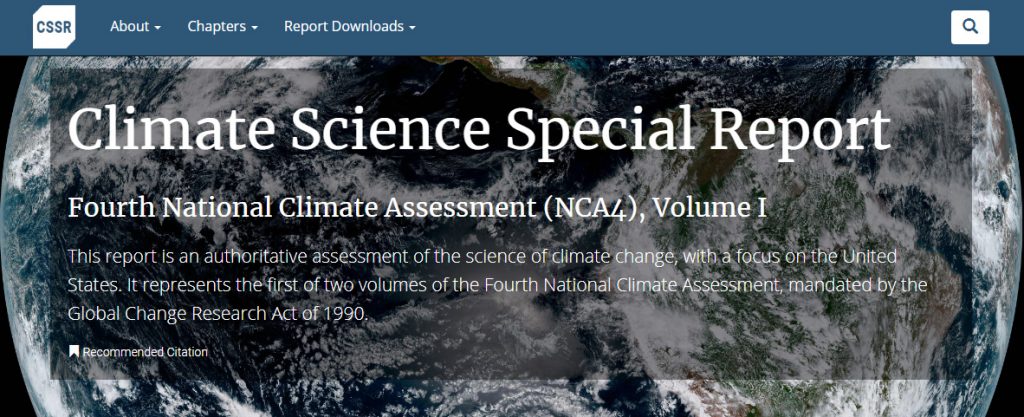The image features a sophisticated interface with a grayish-blue border at the top. Prominently displayed within a white box is the acronym "CSSR." Adjacent to this, a navigation menu includes drop-down options labeled "About," "Chapters," and "Report Downloads." Positioned on the far right is a white square icon with a magnifying glass, signifying a search function.

Beneath this interface, the picture transitions to an awe-inspiring view of Earth from space, capturing the intricacies of the Earth's clouds, oceans, and continents from high above the atmosphere. At the top of this celestial image, large, bold white text prominently declares "Climate Science Special Report." Below this, slightly smaller bold white text reads "4th National Climate Assessment, NCA4, Volume 1." Further down, in plain white text, it elaborates: "This report is an authoritative assessment of the science of climate change with a focus on the United States. It represents the first of two volumes on the 4th National Climate Assessment mandated by the Global Change Research Act of 1990."